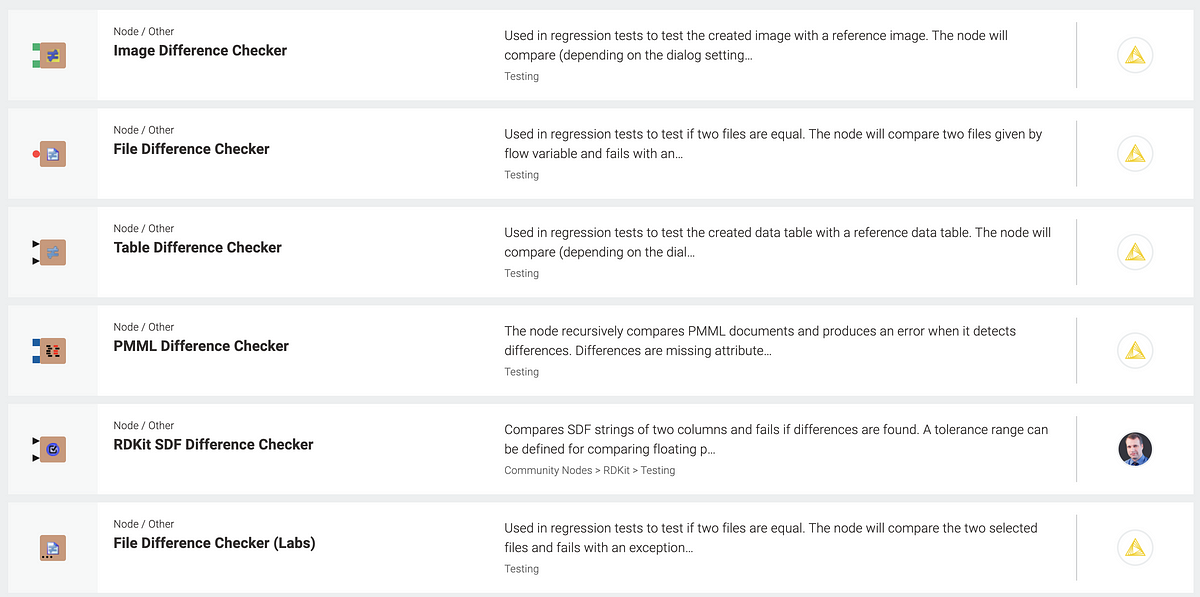---

**Screenshot Description: Detailed Captions of Various Nodes for Regression Testing**

This screenshot is a partial view of an unknown web page, detailing several sections related to different types of nodes used in regression testing. The sections listed are as follows:

1. **Node / Other Image Difference Checker**:
   - Purpose: Used in regression testing to compare a created image with a reference image.
   - Function: This node will compare images based on dialog settings to detect differences.

2. **Node / Other File Difference Checker**:
   - Purpose: Used in regression testing to determine if two files are equal.
   - Function: This node compares two files specified by a flow variable and fails with an exception if differences are found.

3. **Node / Other Table Difference Checker**:
   - Purpose: Used in regression testing to compare a created data table with a reference data table.
   - Function: The node will compare tables based on dialog settings to detect discrepancies.

4. **Node / Other PMML Difference Checker**:
   - Purpose: To recursively compare PMML (Predictive Model Markup Language) documents.
   - Function: The node produces an error when it detects differences in attributes or structures within the PMML documents.

5. **Node / Other RDKit SDF Difference Checker**:
   - Purpose: Compares SDF (Structure-Data File) strings across two columns.
   - Function: Fails if differences are found, with an option to define a tolerance range for comparing floating-point values.

6. **Node / Other File Difference Checker (Labs)**:
   - Purpose: Used in regression testing to verify the equality of two files.
   - Function: This laboratory version of the file difference checker compares two selected files and raises an exception if differences are observed.

These nodes are categorized under "Community Nodes" and further grouped under "RDKit" with a focus on testing various data and metadata artifacts to ensure consistency and accuracy in system regression tests.

---

This detailed description provides clarity and context for each node's purpose and functionality as documented in the screenshot.